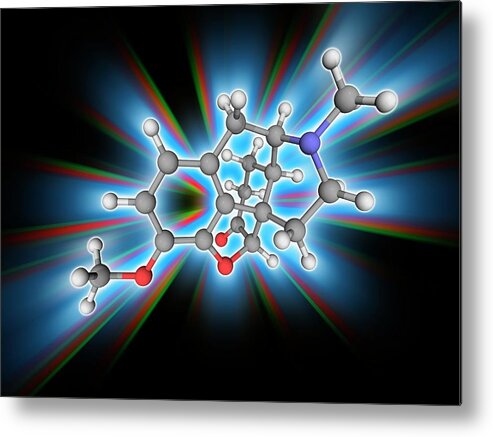This image is a highly detailed illustration of a molecular structure, characterized by white balls representing atoms and cylindrical grey bonds connecting them to form diverse geometrical shapes, including hexagons. The structure appears random yet scientifically precise, with distinctively colored atoms—white, red, orange, and others—interconnected with grey bonds. Set against a stark black background, the scene is illuminated by a vibrant light effect that radiates in streaks of green, blue, and red from the center, giving it a one-point perspective and a sense of dynamic energy. The illustration, reminiscent of something you might find in a science textbook, emphasizes the scientific and educational value of the molecular depiction.